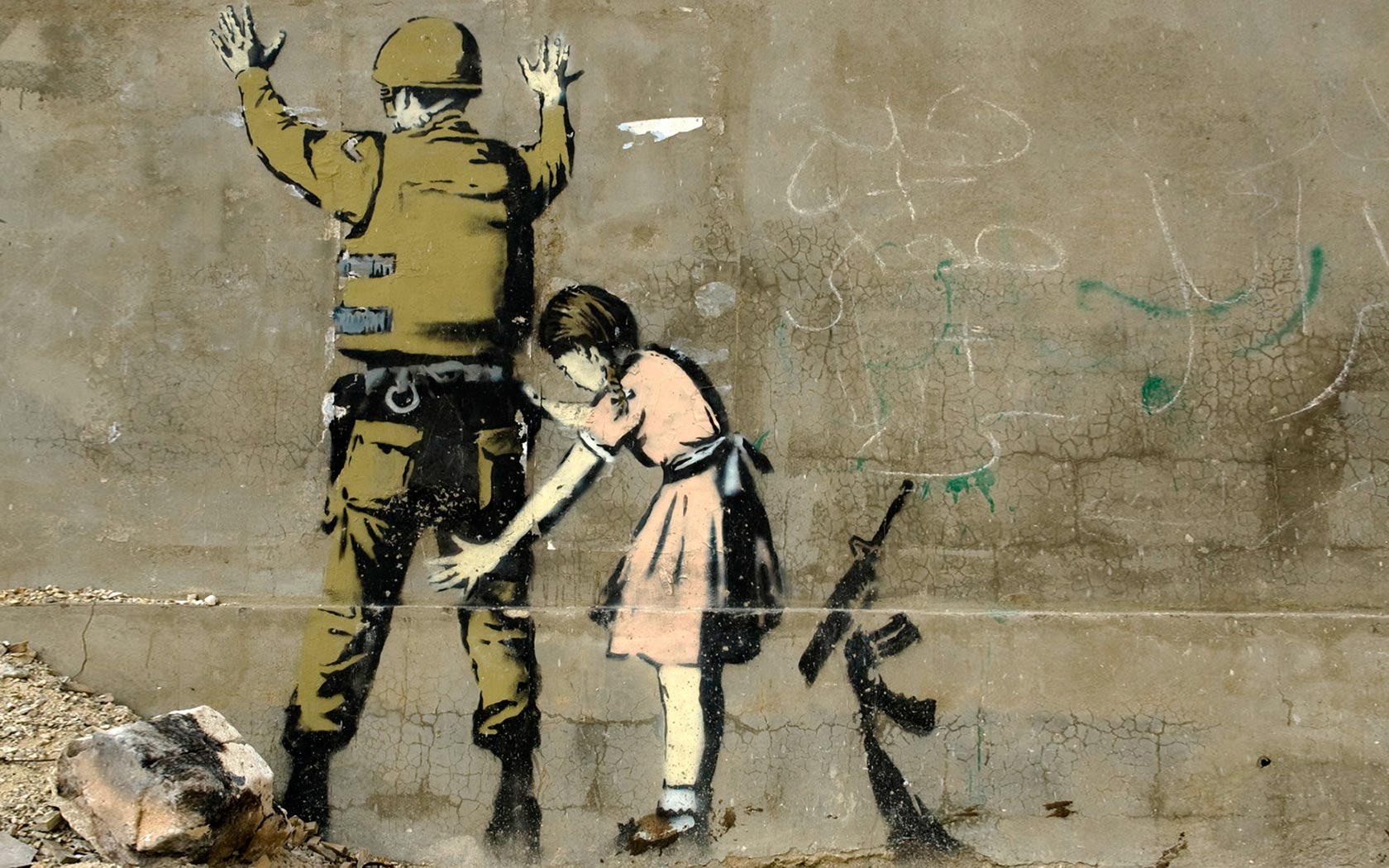The image is an outdoor mural, likely a Banksy piece, stenciled onto an old, weathered wall with cracks and water stains. The wall itself is a mix of gray and brownish colors and contains spray-painted graffiti in a different language, as well as some green spray-painted areas. The mural depicts a scene centered towards the left of the horizontal rectangle, where a soldier in an olive drab military uniform, including a bulletproof vest and helmet, stands with his hands raised against the wall. His position suggests submission as if being frisked. A young girl with brown hair in pigtails is wearing a salmon-colored dress with a white sash belt. She is patting down the soldier, one hand on his hip and the other just below his knee. Next to the girl, there is a dismantled assault rifle visible on the wall. The primary colors used in the mural are peach, army green, gray, black, white, brown, and beige.